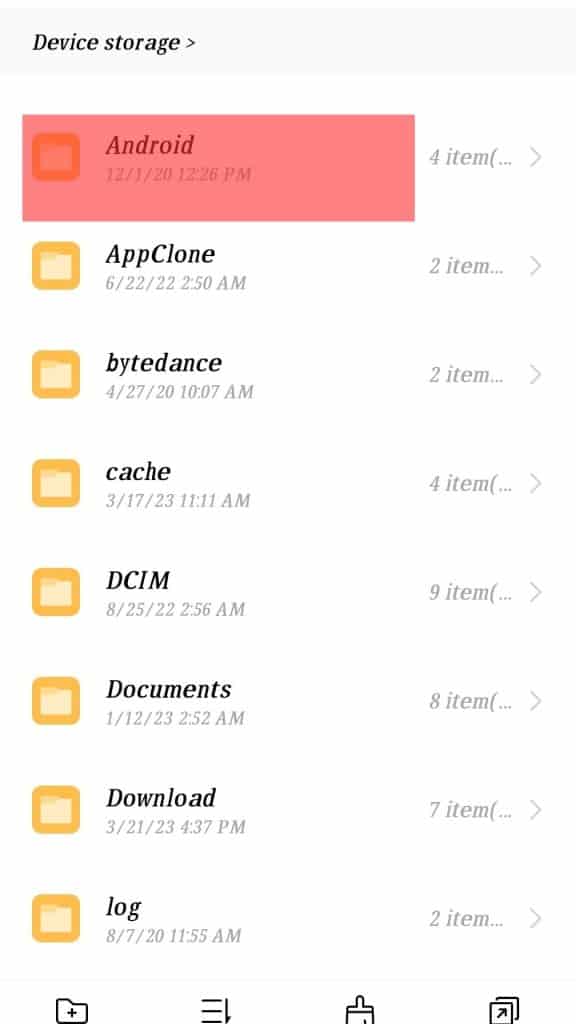The image displays a graphical user interface of an Android device's file storage system on a white background within a gray rectangle. The interface is highlighted in red and features several file folders on the left side. To the right, each folder is accompanied by specific details as follows:

- **App Clone**: Contains 2 items...
- **BYTE Dance**: Contains 2 items...
- **Cache**: Contains 4 items...
- **DCIM**: Contains no items...
- **Documents**: Contains 8 items...
- **Download**: Contains 7 items...
- **Log**: Contains 2 items...

Additionally, there is a file folder with a "+" symbol indicating the ability to add new items. The interface's design includes three lines resembling half of a down arrow and a paintbrush icon, possibly representing additional options or tools for file management.